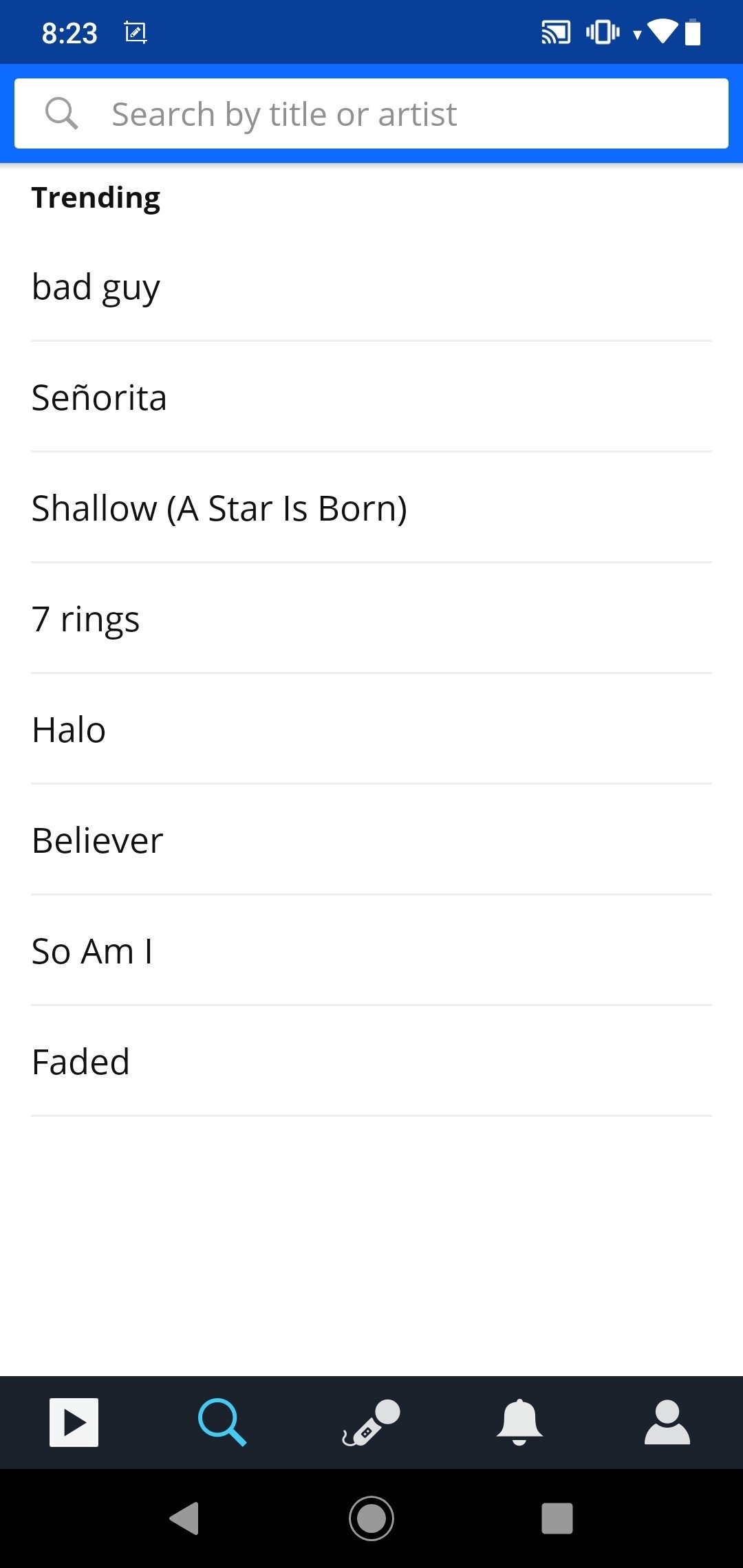A smartphone screenshot captures a music app's search feature in a rectangular format, with its longer sides running horizontally. At the top of the screenshot is a dark blue banner spanning the width of the image. On the left side of the banner, the time is displayed as "8:23." On the right side, there are several icons: a simulcast symbol for sharing the screen on a larger display, a vibrating phone icon, a conical white signal strength indicator, and a fully charged white battery icon.

Just below this banner is a search bar, which is a white rectangular box set against a light blue background. Inside the search bar, grey text prompts the user with "Search by title or artist."

The main portion of the image features a white background with multiple lines of black text organized in a list format. The list begins with "Trending," followed by a series of popular song titles separated by thin grey lines. The songs listed are: "Bad Guy," "Señorita," "Shallow (A Star Is Born)," "7 Rings," "Halo," "Believer," "So Am I," and "Faded." Each song title is distinctly separated by a thin grey line, visually organizing the trending search results within the app.